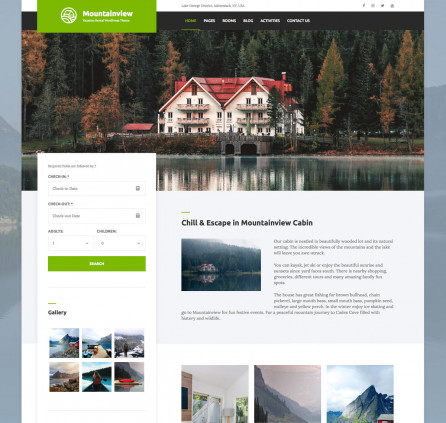**Descriptive Caption:**

The screenshot captures a webpage of an undisclosed website with a small, unreadable font. A green rectangle featuring white text houses a logo and possibly the website’s name, beginning with an 'M.' To the right, a vertical menu bar is present. Below the menu is a sizable photograph of a three-story lake house with a red roof, surrounded by a dense forest, indicating its secluded nature by the lake. A prominent heading reads "Chill and Escape in Mountain View Cabin," accompanied by another image likely showcasing the said cabin, followed by descriptive text. Beneath this section, a row of three smaller photos is displayed, depicting two external and one internal view of the cabin. On the left of the page, filtering options are available for user input, culminating in a green search button.